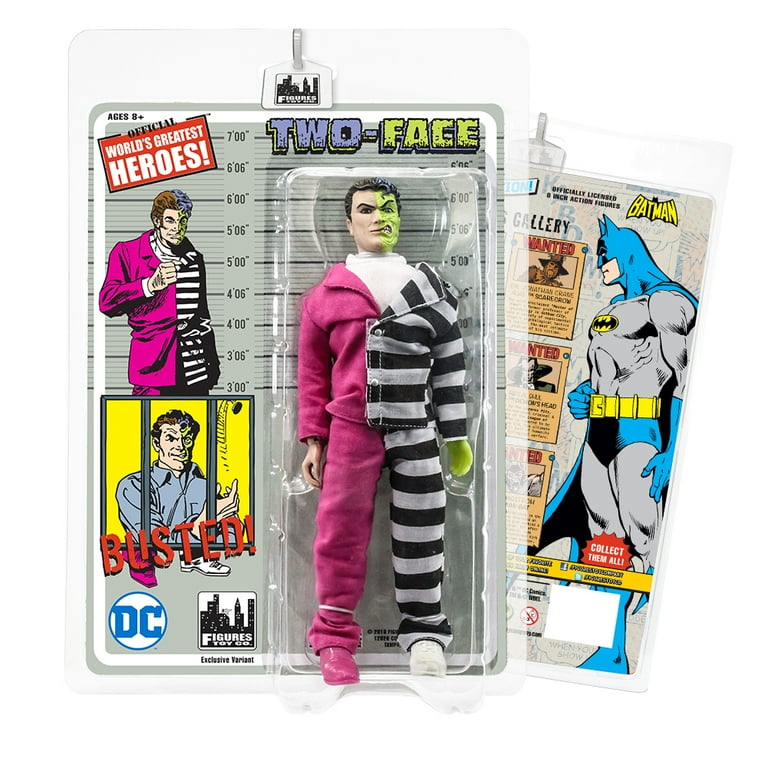The image showcases a DC Comics action figure of the Batman villain Two-Face, presented against a white background. The packaging features a plastic bubble highlighting the Two-Face figure, with a gray cardboard insert behind it. Two-Face is distinctively portrayed with half of his body clad in a pink suit, complete with a pink shoe, and the other half in a black and white striped prison uniform, including a white shoe. Notably, the left side of his face appears as normal Caucasian skin, while the right side is a striking bright green with severe facial scarring, exhibiting an open jaw and a curled eyebrow beneath black hair.

The packaging is adorned with vibrant branding elements: a red box with white text reading "Official World's Greatest Heroes" and the hero's age recommendation ("age 8 plus"), along with a blue and white circle featuring the DC logo. Additionally, a graphic shows Two-Face standing against police height measurement boards, and another detail displays him behind bars with the caption "Busted."

The rear of the packaging glimpsed on the right side of the image features an illustration of Batman in his classic blue and gray suit with a yellow belt and the Batman logo emblazoned on his chest. This compelling combination of visual and textual elements underscores the intricate design and thematic context of this collectible figure.